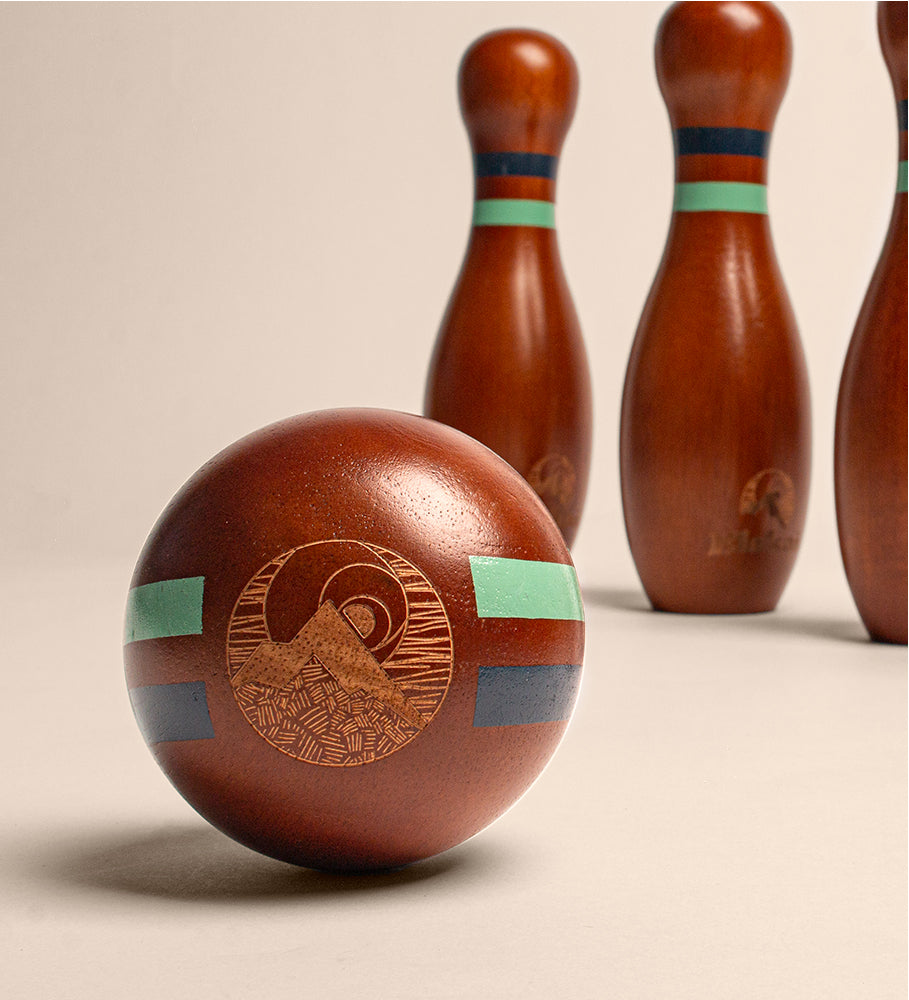In this detailed photograph, you see a set of artistic, high-end wooden bowling equipment. Three bowling pins, each adorned with two color stripes — a light green teal and navy blue — encircle their necks and feature intricate carvings at their bases. The forward object in the image is a wooden bowling ball, its size resembling that of a slightly oversized softball. This ball is decorated with an elaborate design showcasing a mountain and either a moon or a sun. Both the pins and the ball share a reddish wood hue, emphasizing their matching nature. The whole setup exudes an Asian-inspired aesthetic, suggesting it could be part of a luxurious, private bowling alley setup, indicative of high craftsmanship and old-world charm. There are no text elements visible in this elegant and intricately detailed photograph.